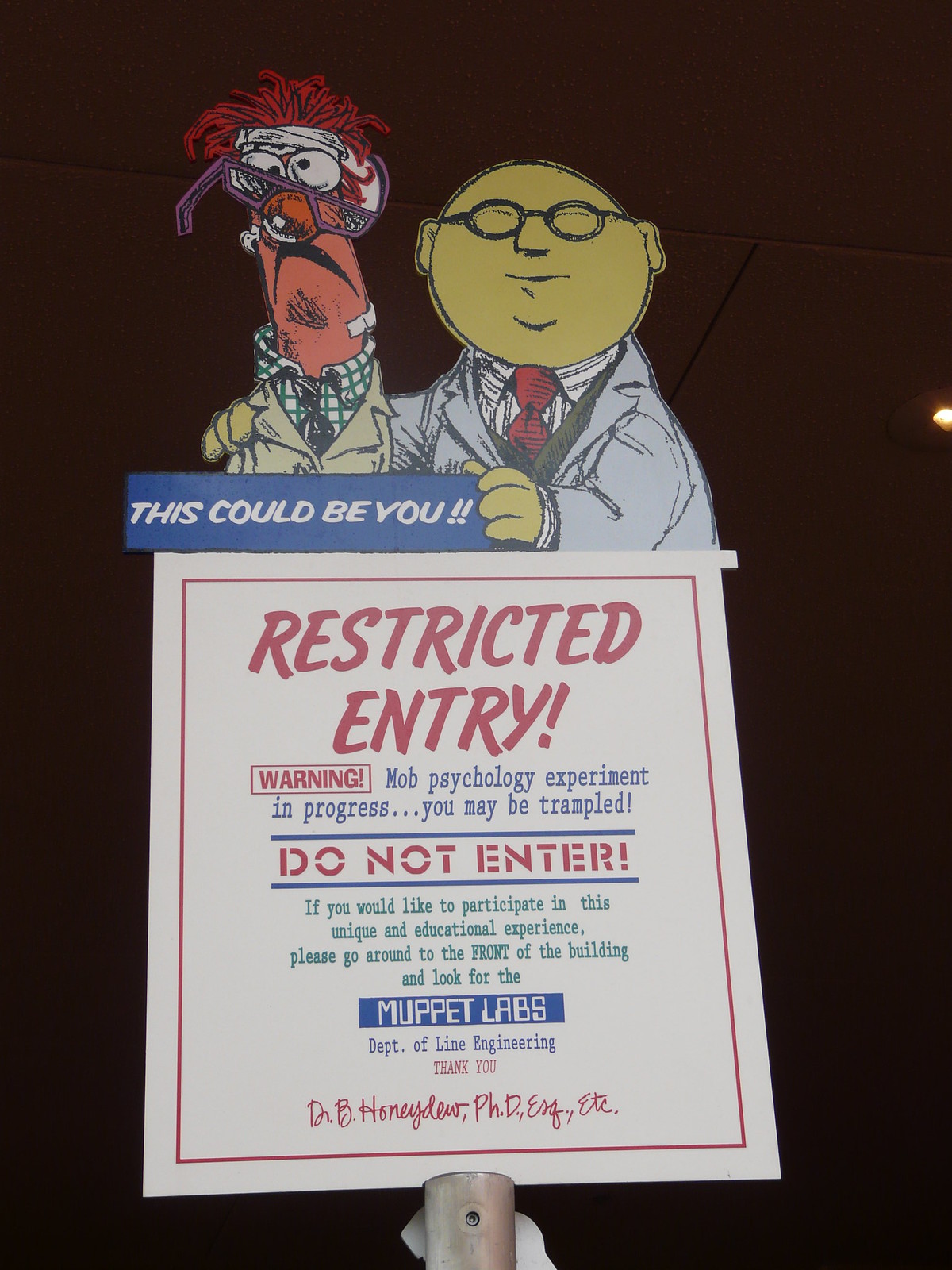Indoors in low lighting, a flash illuminates a sign prominently featuring the Muppets, set against what appears to be a ceiling in the background. The sign is made of cardboard with an off-white hue, topped by images of two distinct Muppet characters. One Muppet, with orange skin and dreadlock-like red hair, looks disheveled in a trench coat over a checkered dress shirt. He appears to have had a rough day. Beside him, a bald, green Muppet with thick glasses, dressed in a white shirt and red tie, resembles a doctor holding a blue sign that reads, "This could be you."

The sign itself has a lower section with various colored text on a white background. In red lettering, it states "Restricted Entry," followed by a blue warning: "Mob psychology experiment in progress. You may be trampled." Then, in red again, it warns, "Do not enter," followed by green text: "If you would like to participate in this unique and educational experience, please go around to the front of the building and look for the Muppet Labs Department of Line Engineering." The message concludes with a bright blue background and white lettering, reading "Thank you." At the bottom, there's a red-inked signature from "Dr. B. Honeydew, Psychology, etc."

This elaborate and colorful sign promises interaction with the Muppet Labs' whimsical educational experiment, emphasizing a mix of humor and caution.